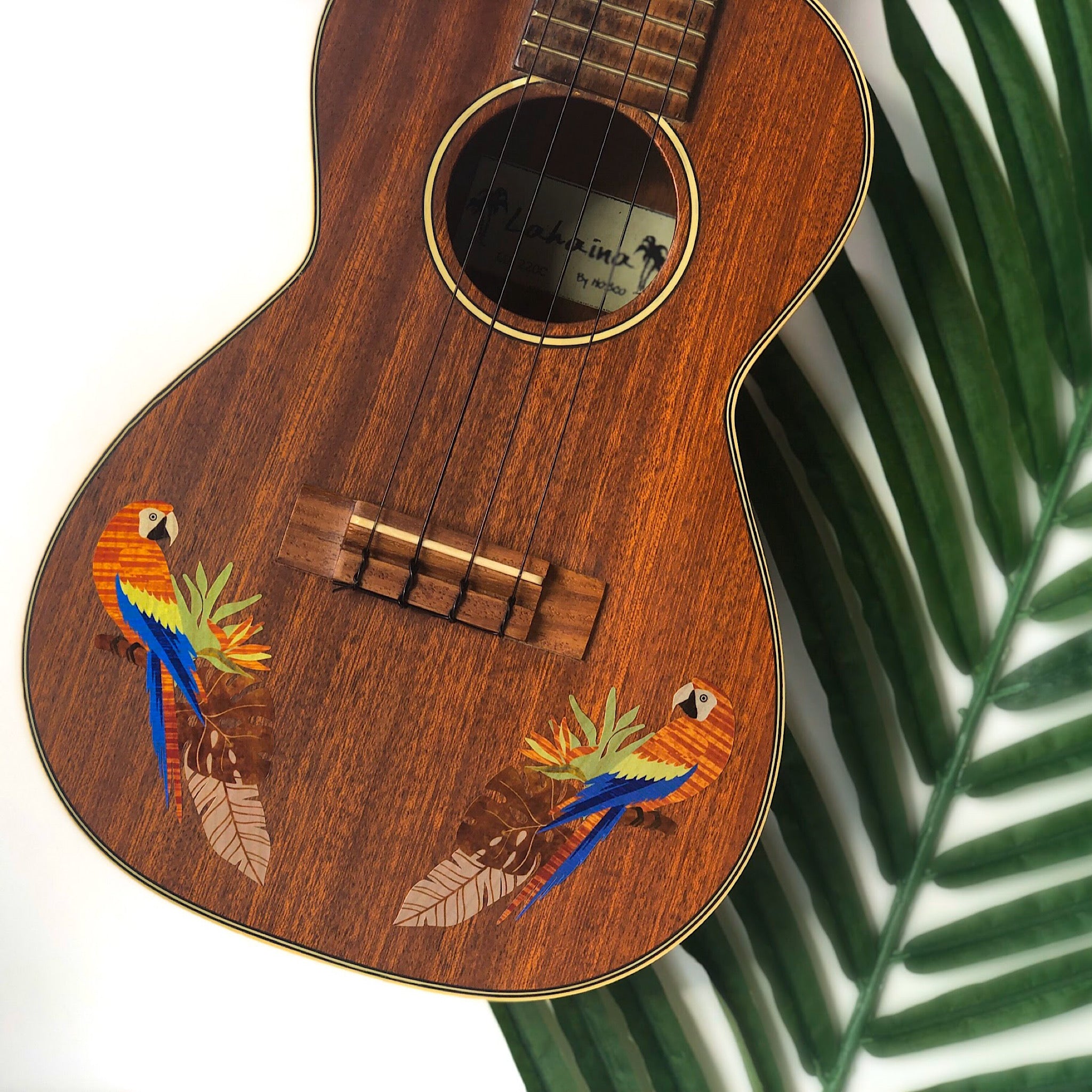This photograph features the intricately detailed body of a dark-stained, four-string ukulele, prominently displayed against a plain white background. The ukulele is adorned with two artistically carved parrots on each side of its lower section, each crafted from a lighter wood. The parrots have small, expressive faces painted in black and white, with vivid blue and green feathers. The birds are perched on a branch with a lush design of leaves; the lower leaves are carved in a dark wood stain resembling a monstera leaf, while lighter foliage patterns embellish the area beneath. The ukulele, positioned at an angle, rests gracefully on a green palm frond that spans the right half of the image. The opening under the neck reveals a shadowed stamp inside that reads "Kahania," although the full text remains obscured. This beautifully composed photograph captures the harmonious blend of nature-inspired design and craftsmanship.